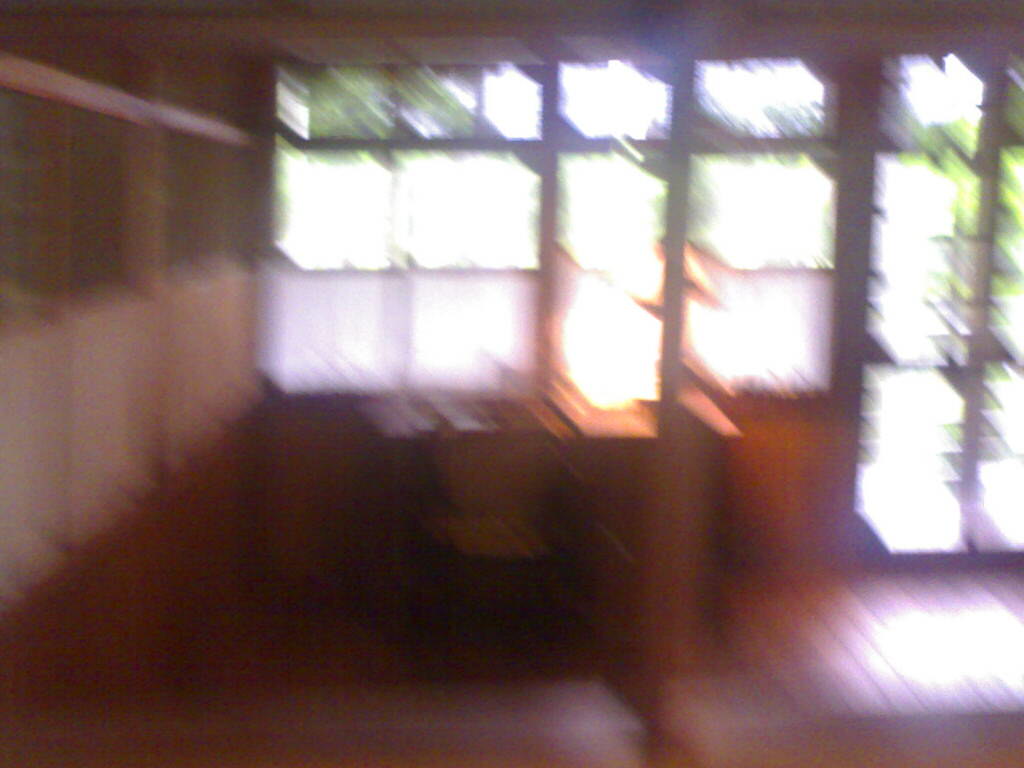This very blurry image depicts the interior of a home, where the central focus is a series of patterned windows that dominate the wall. These windows are primarily divided into four panes each, allowing bright sunlight to stream through. Above these larger windows is a smaller rectangular window featuring two panes side by side. Adjacent to the windows, a door with long, vertical rectangular panes also allows light to penetrate the space. The walls and furniture, including a rectangular desk and a brown chair, are crafted from a bright reddish-brown wood, matching the hardwood flooring that takes on a light to medium hue. On the left side of the image are shelves or cabinets that exhibit a brown base and a white upper section, though the extreme blurriness obscures finer details. Sunlight reflecting off the floor enhances the warm, illuminated atmosphere. Outside the windows, green leaves from trees can be vaguely discerned, contributing to the room's inviting and natural ambiance.